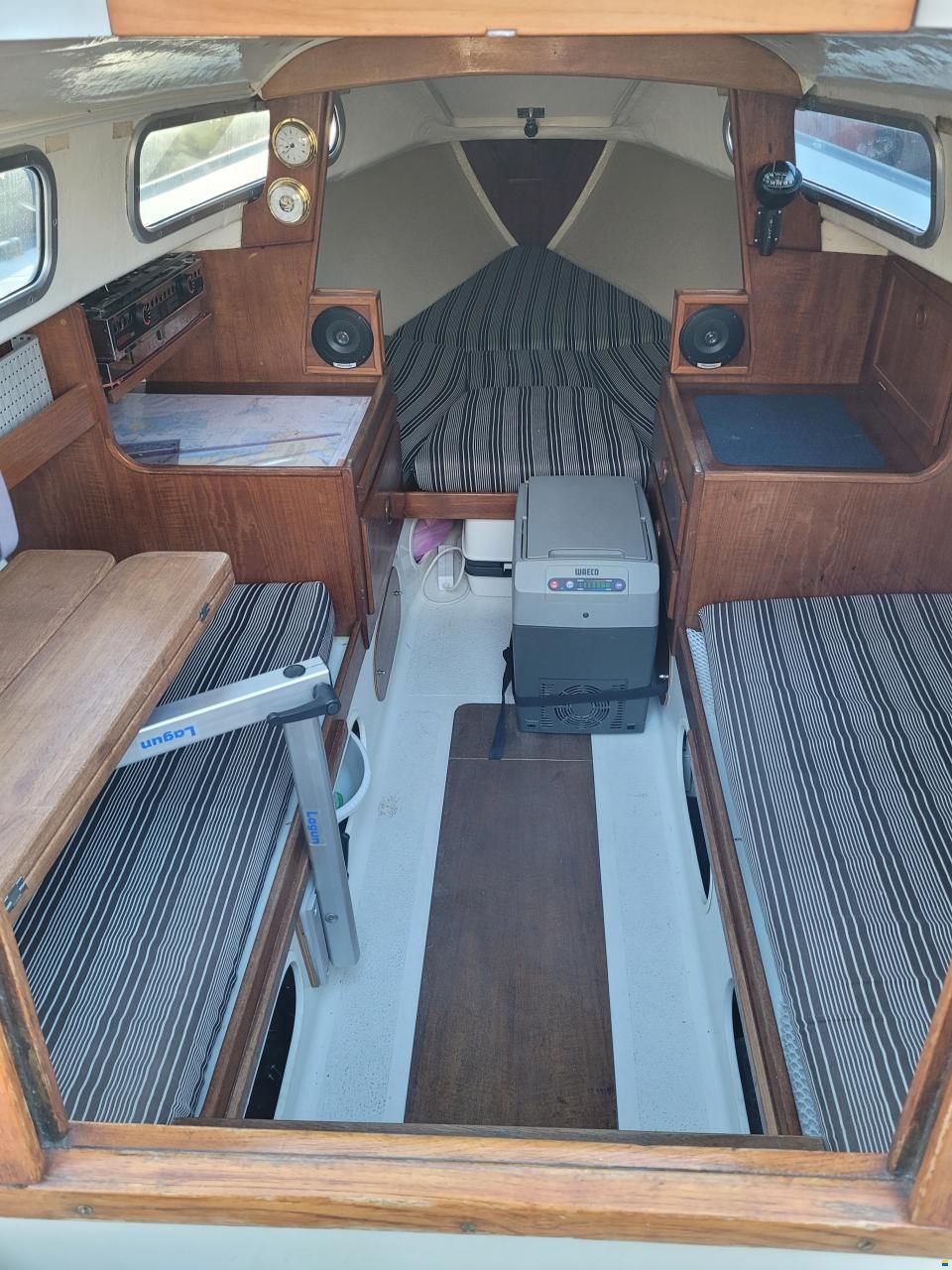This vertical photograph captures the interior of a boat's sleeping cabin, characterized by wooden paneling and practical compact design. The cabin contains two fold-out, pinstripe beds affixed to either side, with cushions for added comfort. At the center, there is a small gray box or cooler. Additionally, a wooden bench provides extra seating or storage space. The back end of the room, a nearly triangular section, houses small windows that wrap around, allowing natural light to filter in. This area also features built-in counters and speakers, with some navigation equipment integrated into the walls, ensuring the cabin doubles as a functional lounging and operational space.